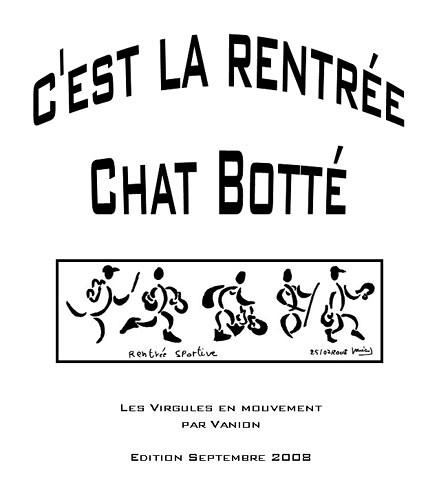The image is a detailed, black and white line art illustration combined with typography and graphic design, set against a white background in portrait orientation. At the top, there is text in French that reads "C'est la rentrée," followed by "Chatebauteille." Below this text, there is a horizontal white rectangle with a black rule around it, containing simplistic stick figure illustrations of five characters. These characters are depicted in various poses, showing animated activities that evoke happiness, such as dancing, jumping, and playing musical instruments like drums and cymbals. Additionally, one figure appears to be holding a sword, another has a hook for a hand, one is riding a scooter, and another has two hooks for hands. Below the rectangle, there is a caption that reads "Rentree Sportive," followed by more French text. The bottom line reads "Edition Septembre 2008." The overall aesthetic combines clean line art with minimalist typography, effectively conveying a lively and joyous theme.